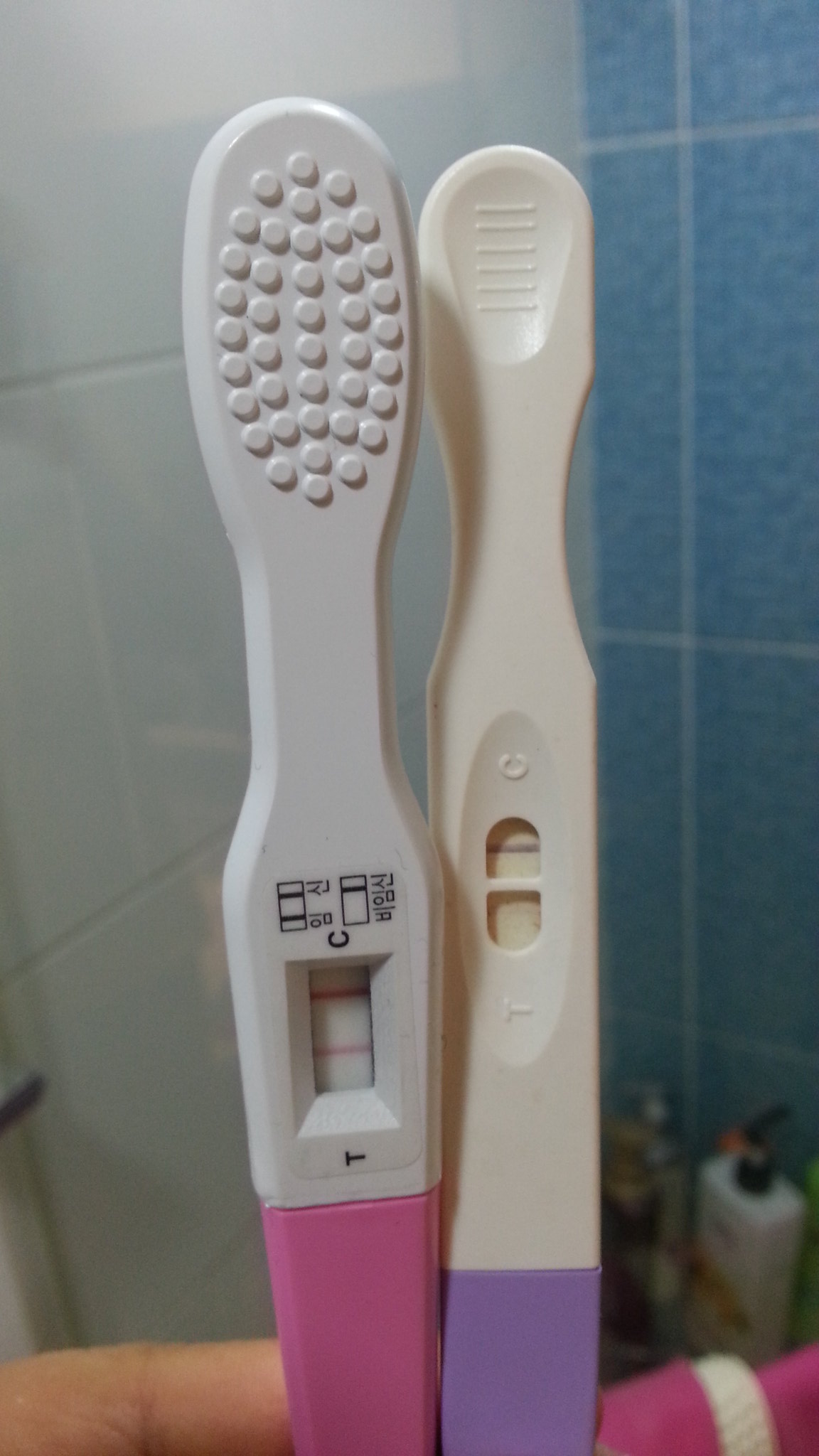In this photograph, two pregnancy tests are being held side-by-side in a vertical position. Both tests are gripped at the side with just a fingertip visible. The pregnancy test on the right features a purple handle. It displays a "T" and a "C" marking, with a single line appearing at the "C" indicator, revealing a negative result. The pregnancy test on the left has a pink handle and bears Japanese characters. This test also shows a "T" and "C" marking, but with two red lines, one at each marker, indicating a positive result. The top part of the test on the right has a textured grip with linear patterns, while the one on the left has circular textures for improved grip.

The setting appears to be a shower, evidenced by the blue tiles on the right and white tiles on the left. On the floor, there are two blue shampoo bottles, further confirming the bathroom environment.